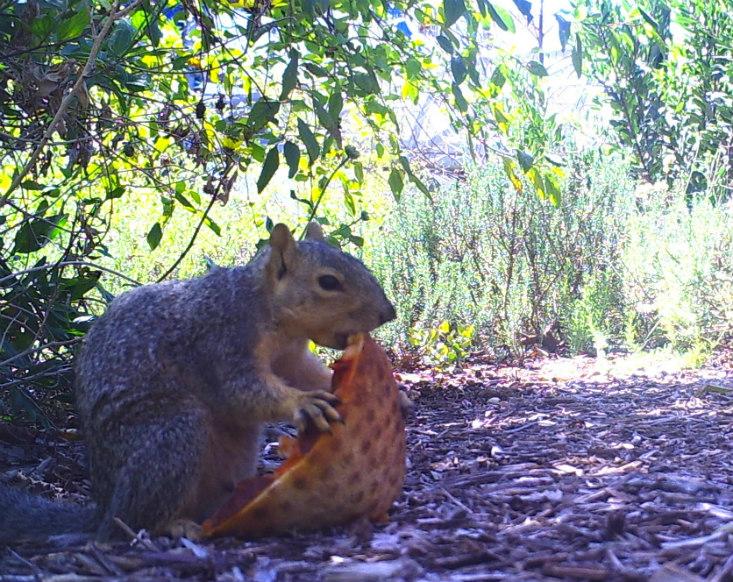In this detailed outdoor image taken in the daytime, a brown and grayish-brown squirrel is prominently featured sitting on mulch amidst a natural setting abundant with greenery, tall grass, and various trees. The sunlight filters through the tree canopy, illuminating the scene and casting shadows. The squirrel, with brown eyes and a tan belly, is perched on its hind legs, holding a triangular slice of pepperoni pizza with both hands. The pizza, offering a clear view of the seared crust, cheese, and pepperoni slices, is being nibbled on by the squirrel, who has the pizza in its mouth. Around the squirrel, fallen leaves and sticks are scattered on the ground, indicating a woodland environment. The squirrel’s bushy tail adds to its distinctive appearance as it enjoys its unexpected meal.